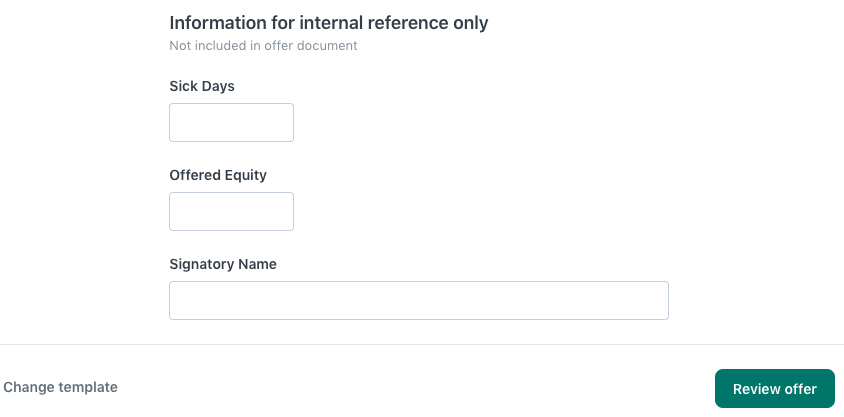This image captures a webpage with a predominantly white background. In the top left corner, approximately two inches from the edge, there is bold black text that reads "Information for Internal Reference Only." Below it, in smaller black lettering, it states "Not Included in Our Document." A small gap follows. The next section features bold black text that reads "Sick Days," with a rectangular input field below it, outlined with a gray border and a white interior. Further down, another bold black heading says "Offered Equity," followed by a similar rectangular input field, both approximately two inches in length. 

Next, another bold black label, "Signatory Name," appears with a corresponding rectangular input field extending to about two inches from the right edge of the page. Directly beneath this, there is a thin gray line stretching across the page from left to right. In the lower-left corner, smaller black text spells out "Change Template." Directly opposite, on the right side of the page and below the gray line, there is an aqua green tab. This tab contains the white capitalized letter "R" in the word "Review," followed by the word "Offer."